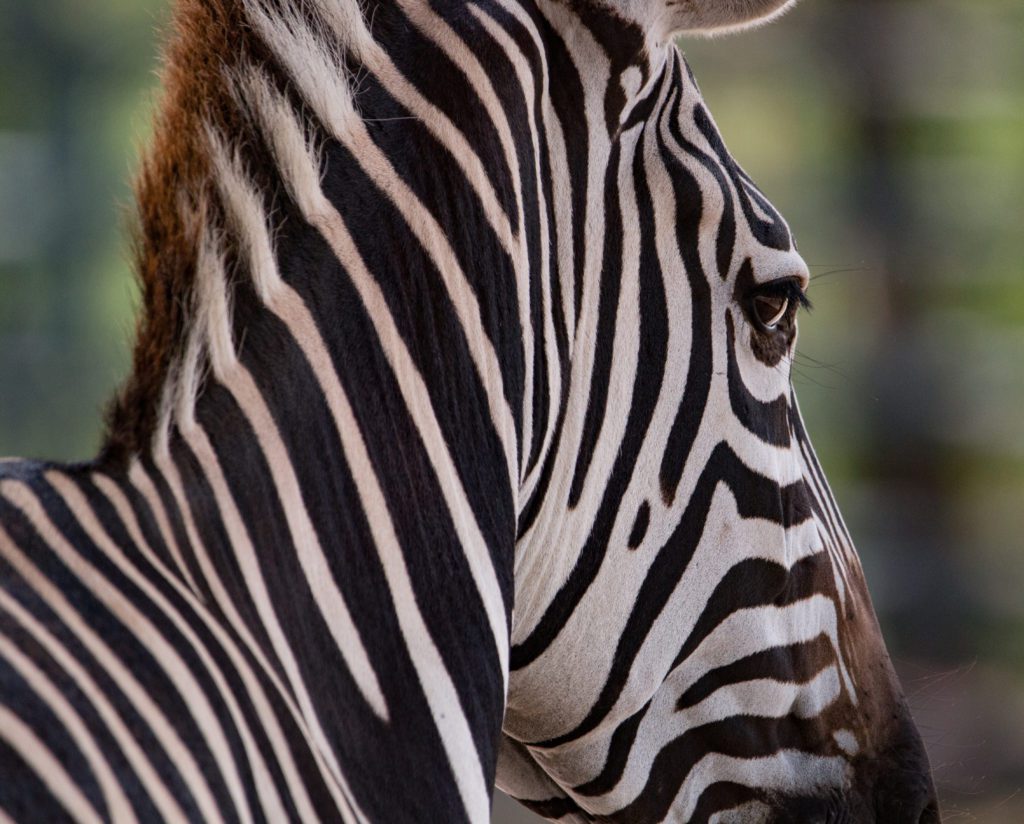This high-quality, zoomed-in photograph captures a zebra from a right-side perspective, with a blurred green background emphasizing the animal as the main subject. The image prominently features the zebra's right eye, which is black with thick short lashes and some longer sparsely spaced ones. The zebra appears to be looking back towards the photographer. Only portions of its nose and chin are visible, with the muzzle being black and a dark brown patch just above it. The distinct black and white stripes cover the zebra’s head and neck, while part of its mane and ears are also seen. The detailed focus highlights the intricate patterns and textures of the zebra’s face and neck against a bokeh background.